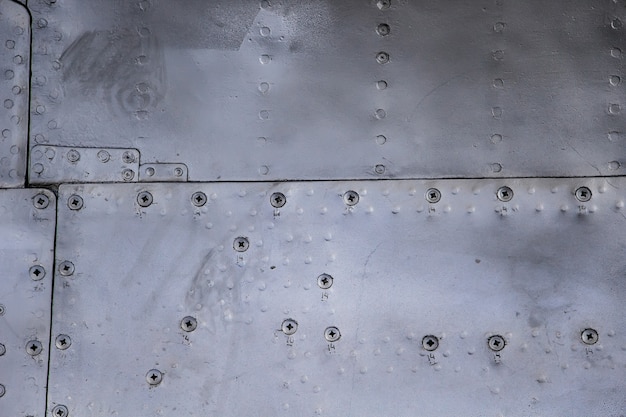This close-up color photograph features the riveted steel panels of either a ship or an aircraft. The metallic surfaces are a gray or silver hue, covering the entire frame with a detailed focus on the rivet patterns. Four primary panels are visible towards the left side of the image, arranged with the bottom panels overlapping the top ones. Along the seams of these panels, rivets are evenly spaced, complemented by several randomly placed rivets on the bottom panel, numbering around seven to nine. Each rivet matches the gray metallic color of the panels. The photograph also highlights various smaller rectangular metal pieces and divots across the panels, suggesting precise tool work. The image reveals subtle weathering on the steel, emphasizing its industrial and potentially aged character. The intricate arrangement of rivets and panels is a testament to the meticulous construction and durability of the metal surface depicted.